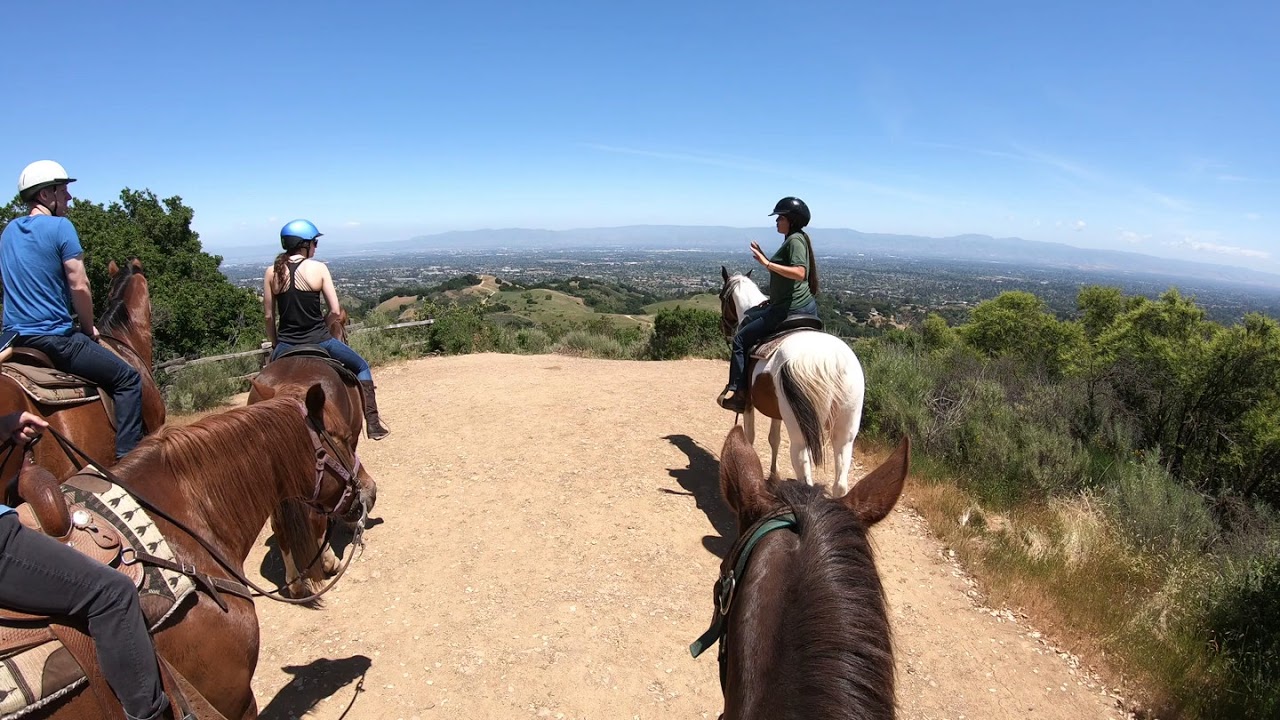The image is a detailed, photorealistic, landscape-oriented photograph taken from the back of a brown horse, likely suggesting that the photographer is also on horseback. The viewer's perspective is slightly elevated, creating a slight downward look, making it appear as though a drone might have taken the photo. The scene captures an outdoor daytime setting under clear blue skies, overlooking a vast scenic vantage point with faint hills and a green, tree-filled plain in the background. 

A broad, light-colored dirt path weaves through the image, with four horses and their riders progressing away from the camera. In the immediate foreground, a brown horse's head is visible just to the right of center. Directly ahead, a white and brown horse carries a rider dressed in a black helmet, green shirt, and blue pants, leading the group. Three more riders on brown horses can be seen to the left, though partially obscured by the image's edge. The rider closest to the group on the left is a man with a white helmet, blue shirt, and blue pants. Another rider ahead of him is a woman wearing a blue helmet, a black tank top, and blue pants, identified by her brown hair tied back in a ponytail.

The path itself is flanked by various vegetation, including grasses and shrubs, with trees lining the left side and shrubs on the right. This wide and slightly winding trail overlooks a distant canyon valley, which is carpeted in green grass and tall trees, with a purple mountain range visible on the horizon. The riders, all equipped with helmets, create a harmonious balance as they traverse this vast and picturesque landscape, blending seamlessly into the natural beauty of their surroundings.